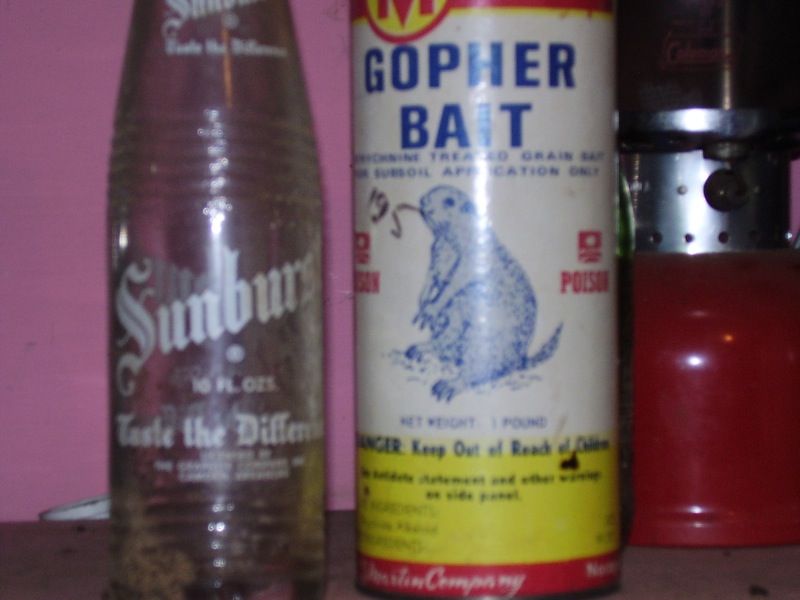In the photograph, three distinct objects are arranged from left to right on a plain wooden table, set against a lavender-colored wall. 

On the left is a slightly blurry, presumably empty container labeled "Sunburst," with text indicating "Taste the Difference" and "10 fluid ounces." Given the context and appearance, it likely once contained some form of sugary juice.

In the middle, there is an old, worn package of "Gopher Bait," featuring a retro design. The package prominently displays warning labels such as "Danger," "Keep out of reach of children," and "Poison," alongside an illustration of a gopher.

On the right, there is a red object resembling a modified tea kettle. It features a silver cap where the lid would typically be located, although its exact purpose is unclear.

Despite the overall blurriness of the image, each item's distinct characteristics provide a glimpse into their diverse backgrounds and potential usages.